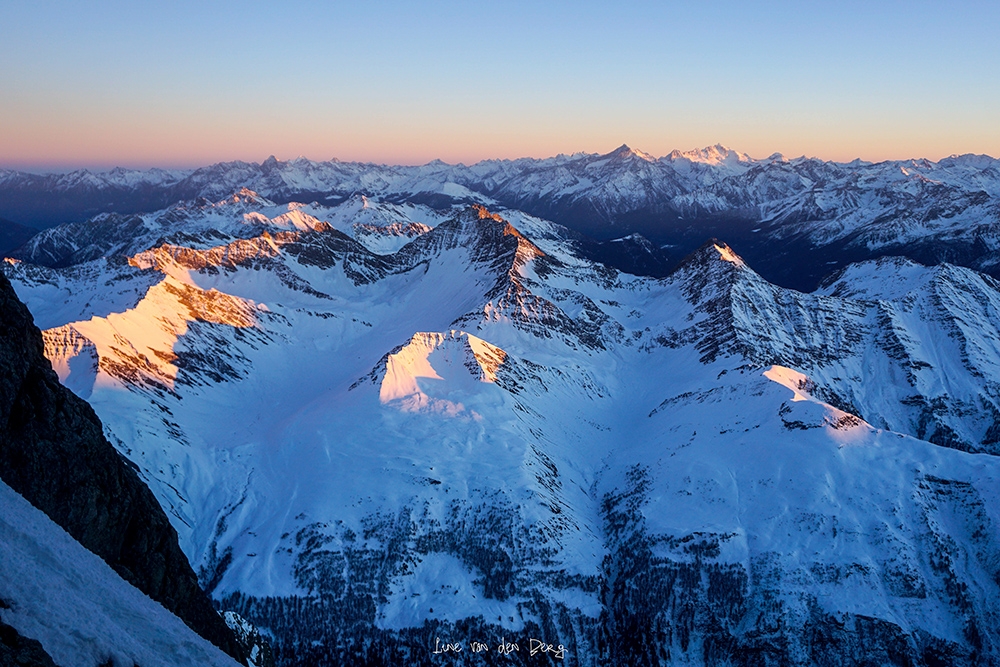This aerial photograph captures a breathtaking winter landscape of snow-capped mountain ridges stretching as far as the eye can see. The peaks are bathed in soft light that suggests either sunrise or sunset, casting a beautiful glow over the snow and creating a striking contrast with the shadows on the slopes. The sky transitions from a light blue to a warm reddish-orange near the horizon, enhancing the serene and majestic atmosphere. The mountains dominate the scene with no visible trees or buildings, only pure, unspoiled nature. In the center bottom of the image, barely visible in faint white cursive text, appears to be an inspirational message, possibly saying "live for the day." The perspective indicates that the photo was taken from a plane flying close to the side of a mountain, offering a stunning vantage point of the rugged and pristine terrain.